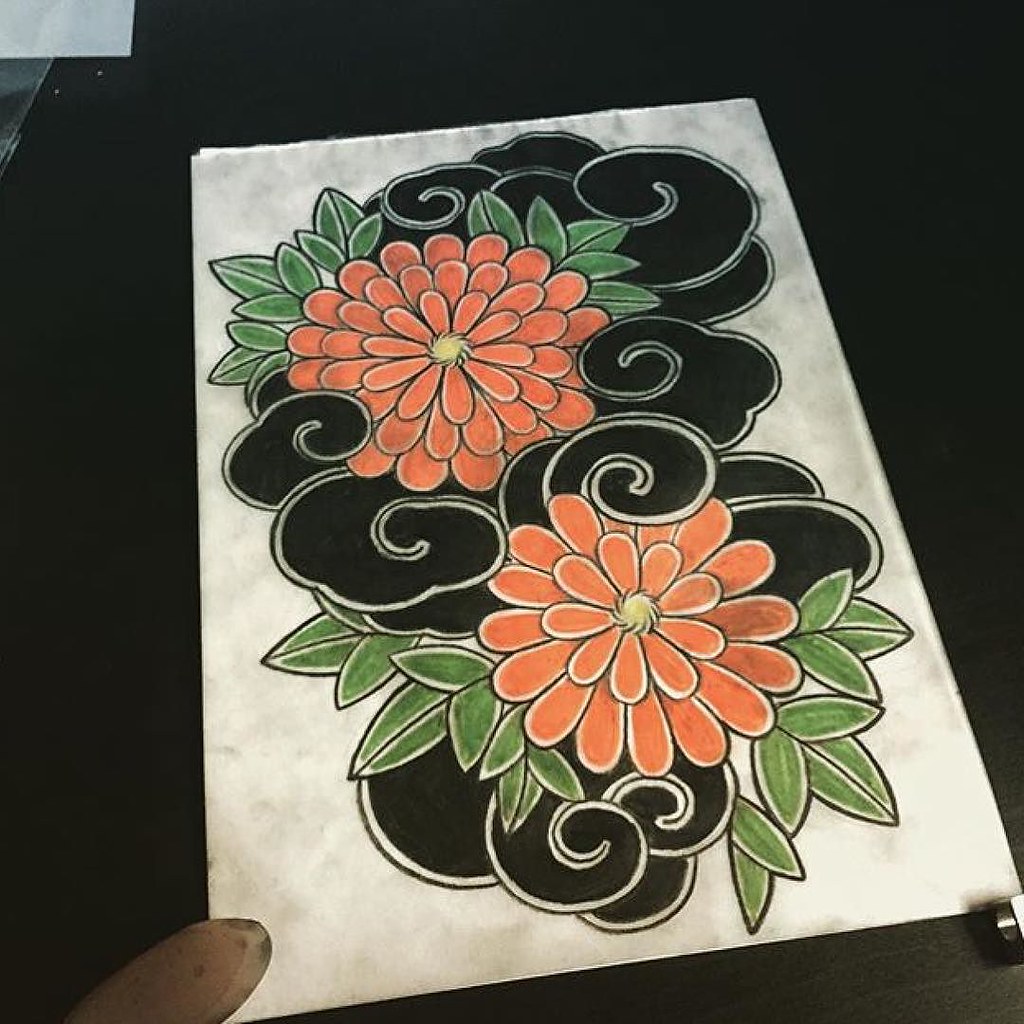This artwork, rendered on a white sketch pad paper, appears to have been created using pastel pens, giving it a chalky texture. Dominated by hues of black, orange, and green, the composition features two large, vividly colored flowers. The top flower boasts three distinct rows of petals with a bright yellow center, while the flower below it has two rows of petals. Both flowers have leaves extending from their base. A background of swirling dark black clouds envelops the scene, weaving between the flowers and leaves, adding a sense of depth and drama to the piece. Smudges of darkness are scattered across the background, enhancing the contrast and making the vibrant colors of the flowers pop even more strikingly.